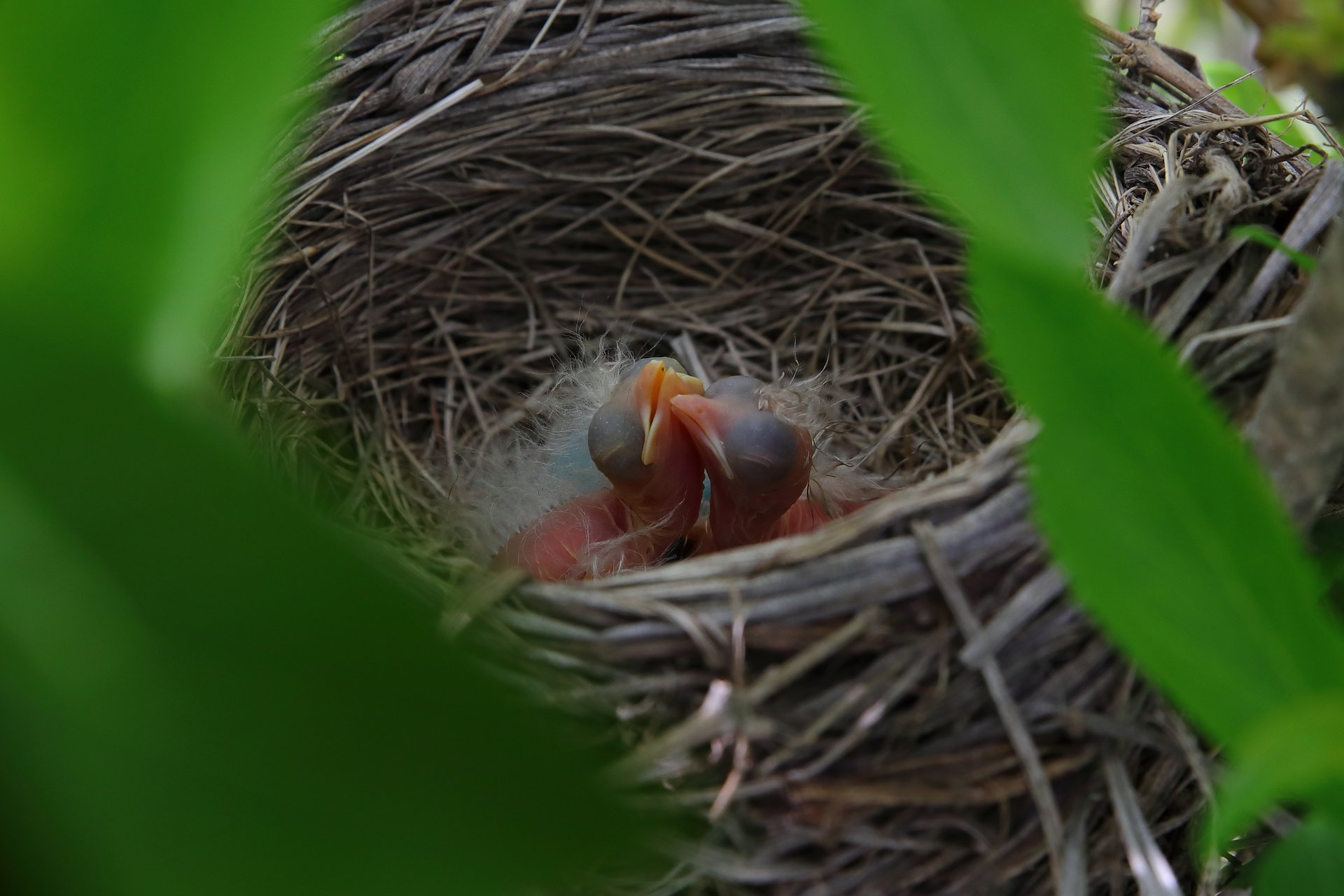This is an extreme close-up photograph of a bird's nest showcasing an intimate and touching moment between two newly hatched baby birds. Nestled in a matted circle composed of straw, pine needles, and small sticks, the nest features a fluffy bottom layer providing comfort for the delicate hatchlings. The baby birds, with their beak against the neck of one another, are lying in a touching embrace, both facing upward. They appear featherless and with closed eyes that look like translucent, gray bubbles, characteristic of their very young age. The bird on the right has a yellow beak with white accents towards the ends, while the one on the left has an orange beak. The nest is surrounded by brown and gray materials and encircled by various leaves, varying from light to dark green, which frame the photograph. In the background, blurred soil and grass create a soft, natural backdrop. This harmonious composition is viewed through the foliage of the tree, with leaves partially obstructing the view from the corners, enhancing the close and protected atmosphere of the image.